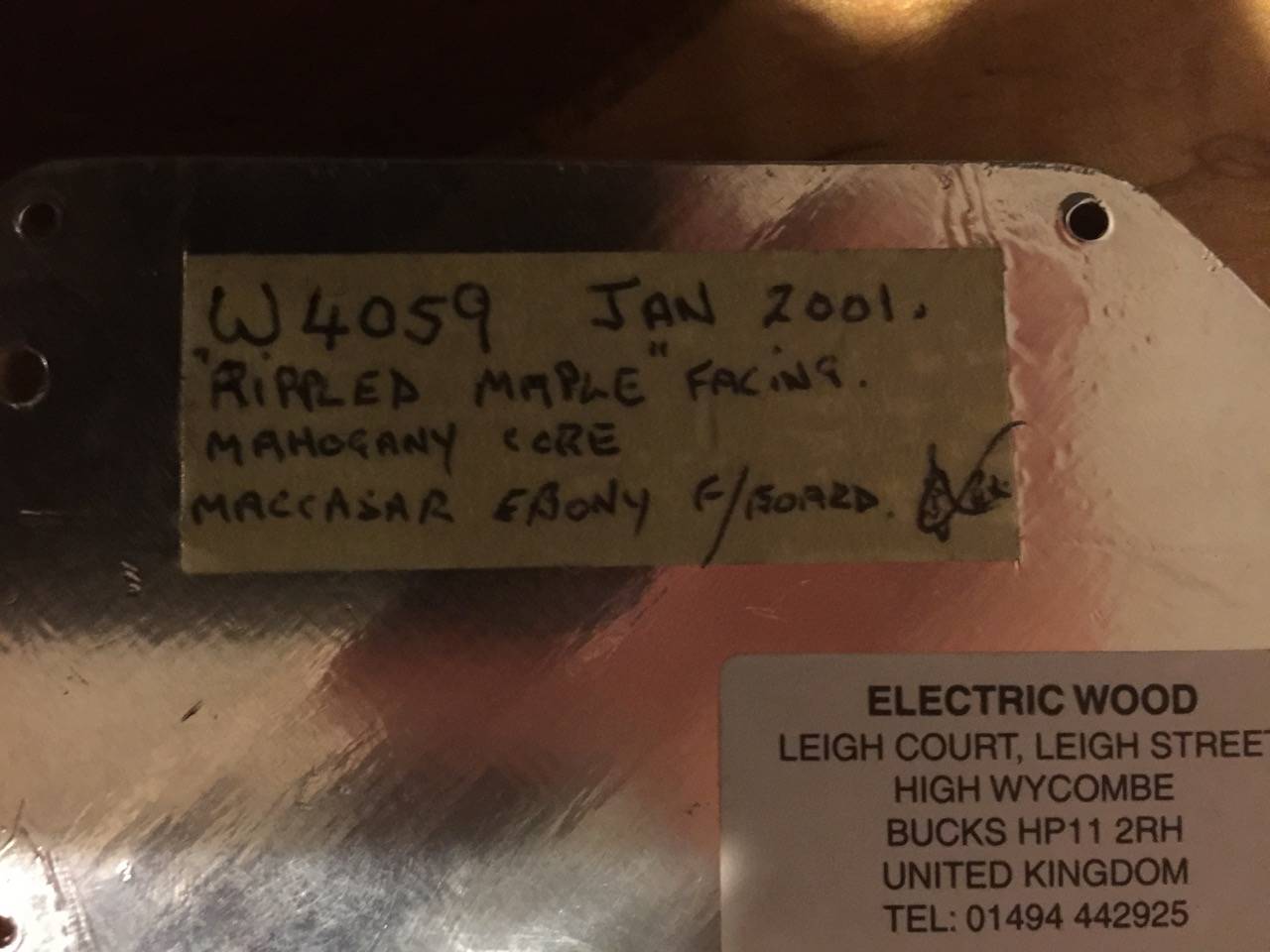The close-up image showcases a metallic, silvery, reflective surface adorned with numerous small holes. On this surface, there is a handwritten label affixed with tape. The label reads: "W4059, JAN 2001" in handwritten text. Beneath this, within quotation marks, it states: "Rippled maple facing, mahogany core." Below that, it mentions: "Macassar ebony F/board." Toward the bottom right corner, a white printed label can be seen. This label features bold capitalized text reading: "Electric Wood," followed by "Lee Court, Lee Street, High Wycombe, Bucks, HP11 2RH, United Kingdom, Tel: 01494 442925." Reflective elements on the metallic surface, including the faint outline of a person taking the image, add to the visual complexity.